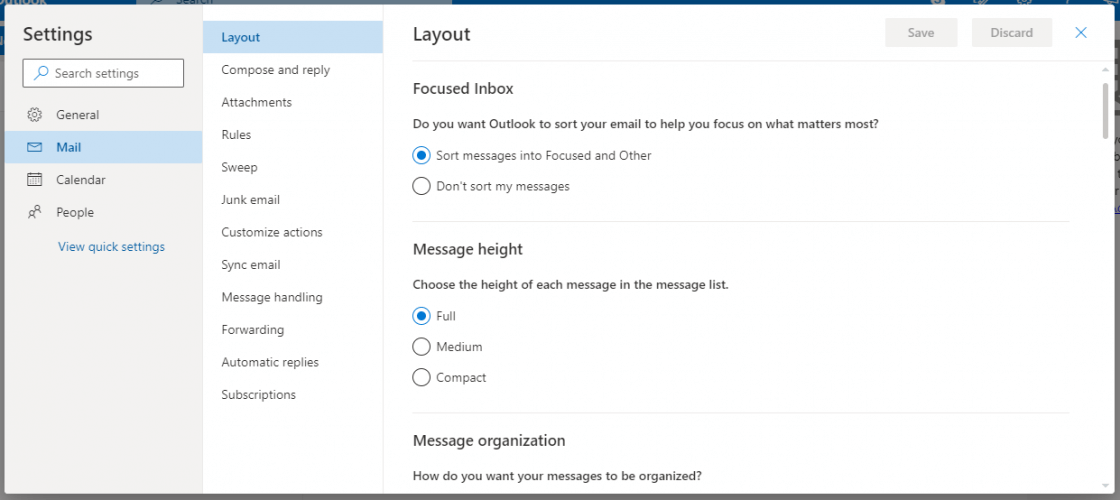**Screenshot of Microsoft Outlook Settings Tab**

The image is a screenshot from the settings tab in Microsoft Outlook. At the top left corner, the word "Settings" is displayed prominently. Directly below it is a search bar labeled "Search settings."

The left sidebar contains a menu with several options, including:

- **General**
- **Mail** (this is highlighted in blue)
- **Calendar**
- **People**

Under the "Mail" category, multiple sub-options are listed, featuring:

- **Layout** (highlighted in blue)
- **Compose and Reply**
- **Attachments**
- **Rules**
- **Sweep**
- **Junk Email**
- **Customize Actions**
- **Sync Email**
- **Message Handling**
- **Forwarding**
- **Automatic Replies**
- **Subscriptions**

The main content area displays the "Layout" tab details, starting with a section on "Focused Inbox." The prompt reads: "Do you want Outlook to sort your email to help you focus on what matters most?" There are two radio button options:

1. **Sort messages into Focused and Other** (this option is selected)
2. **Don't sort my messages**

Below this, there's a section titled "Message Height" with the prompt: "Choose the height of each message in the message list." The options provided are:

- **Full** (this is selected)
- **Medium**
- **Compact**

Next, the "Message Organization" section asks: "How do you want your messages to be organized?" The bottom part of the settings interface shows options to "Save" or "Discard" changes, but these buttons are grayed out. Additionally, there is a blue "X" mark at the far side of the screen.

**Note:** The phrase "Leah, baby" appears in the transcription but seems unrelated to the settings content and could possibly be an erroneous input.